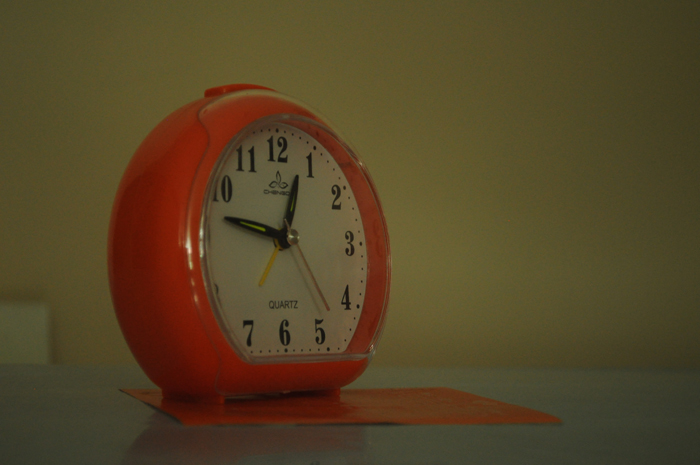In a high-quality, dimly lit photograph, a small square red mat sits close to the foreground on a highly reflective tabletop or countertop, which is positioned against a yellowish blank wall. Atop the mat stands an older-style clock with a circular red plastic body and a glass shield protecting its face. The clock is supported by two small legs, ensuring its stability on the mat. The timepiece features distinct minute, hour, and second hands. Below the number six, the word "Quartz" is clearly visible, while just beneath the number twelve, the clock's brand name and a delicate leafy logo are displayed. The minimalist setting and subdued lighting draw attention to the intricate details and retro charm of the clock, making it the focal point of the composition.